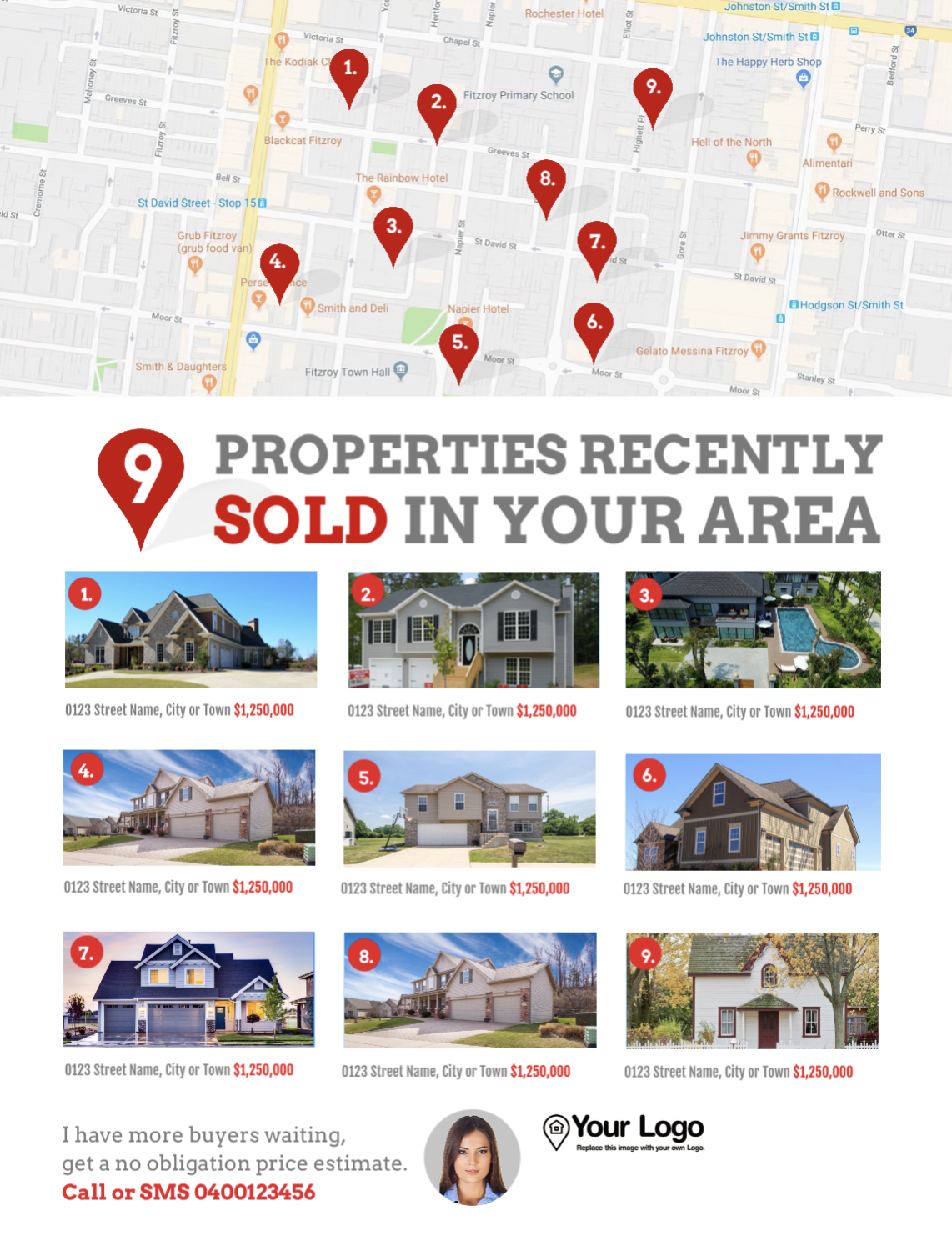The top section of the image features a Google Maps screenshot predominantly displaying gray areas, intersected by white lines and long yellow lines. There are two green areas and nine large, red markers shaped like inverted teardrops, or resembling the shape of hot air balloons—round at the top and tapered at the bottom. Below the map, there is an icon of an inverted teardrop containing the number nine, signifying the quantity of properties.

To the right, text in gray reads "Properties Recently" followed by "Sold in Your Area" in red. Below this, there is a listing of nine upscale homes, each valued at a million dollars or more. The houses generally feature triangular roof designs and appear quite large and similar in structure.

Further down, there's a section encouraging potential sellers with the message "I have more buyers waiting. Get a no-obligation price estimate" in gray, accompanied by a red-colored invitation to call or SMS the number 0400-123456.

On the far right, a circular profile image shows a woman with dark brown hair wearing a blue shirt, looking serious and not smiling. Adjacent to this profile image, the text reads "Your Logo."